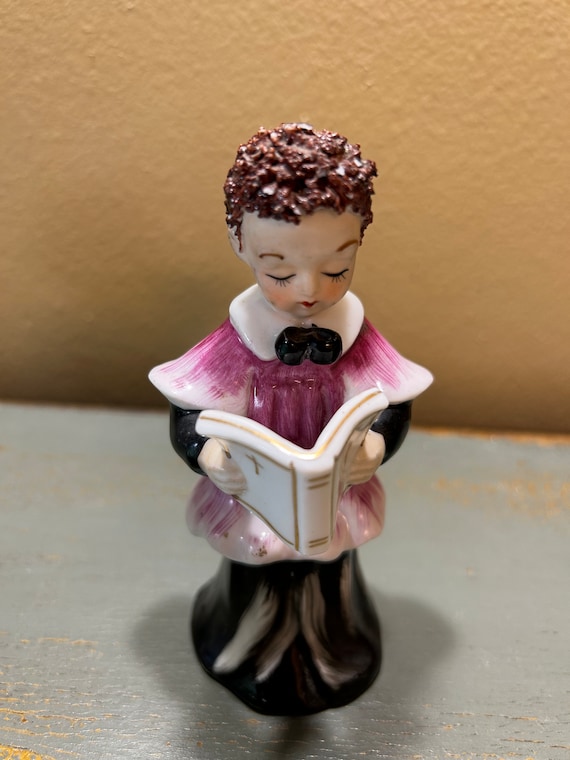This vertically aligned, full-color photograph showcases a small, delicate porcelain figurine carefully staged indoors. The backdrop features a textured yellow wall, transitioning to a chipped, gray-painted wooden tabletop that reveals patches of the wood's natural brown beneath. The figurine portrays a young child with short, curly brown hair, eyes cast downward as if engrossed in reading a small white book adorned with gold outlines and a cross, likely representing a Bible or hymnal. The child, with defined eyelashes and a serene expression, is dressed in a black and white garment with a red lipstick hinting it might represent a girl. The outfit includes a white collar and a distinctive black bow tie. The figurine evokes a sense of reverence as it stands on the worn tabletop, melding simplicity with intricate detailing.